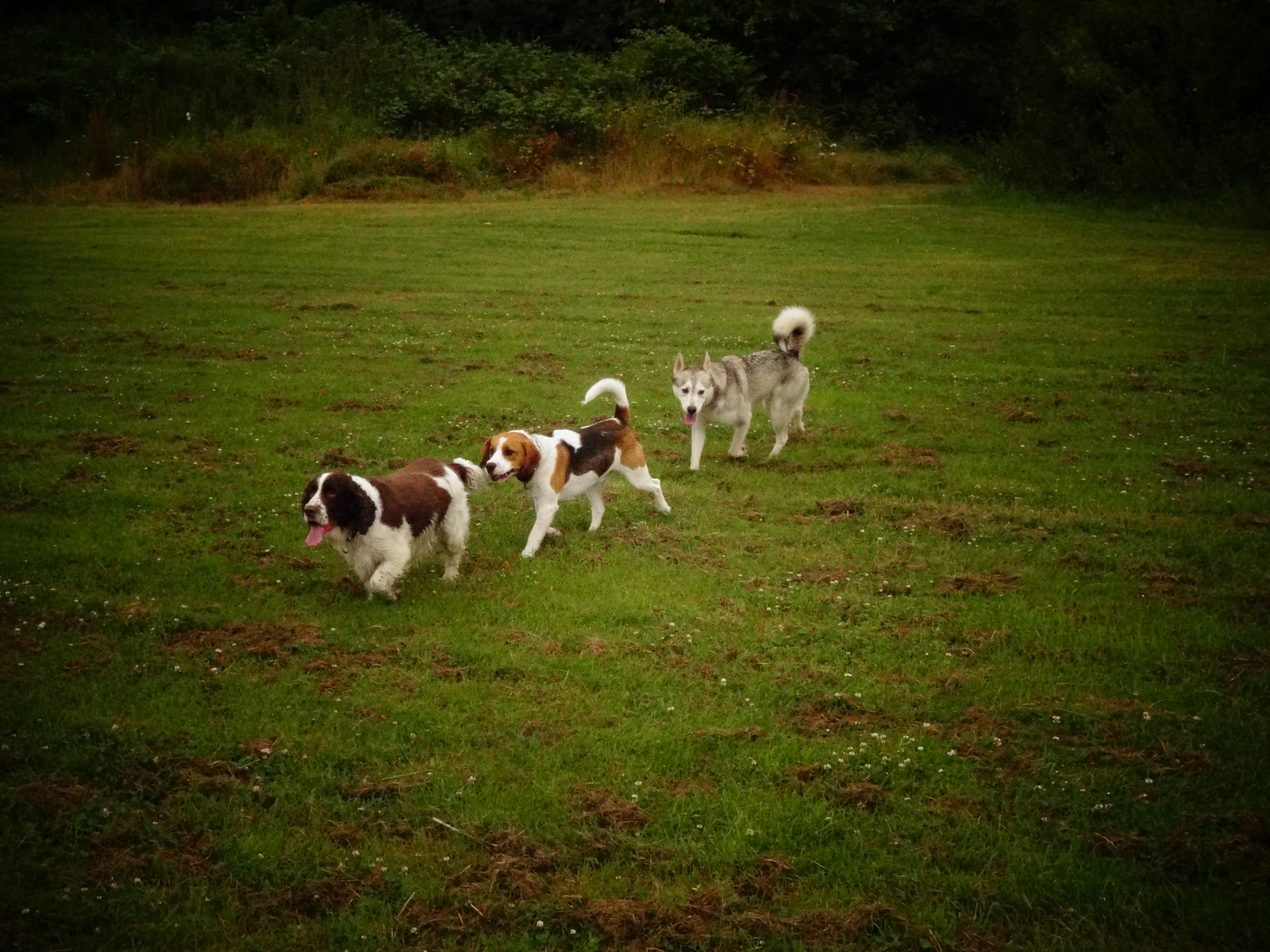In this outdoor photograph, three dogs walk in a diagonal line across a grassy field, with greenery such as bushes and trees in the background. The photo has a dark vignette, making the edges much darker than the center, and overall, the colors are muted and lack vibrancy. The first dog, leading the line, is a heavyset canine with a white body and brown patches on its back and ears; its tongue is hanging out, giving it a cheerful appearance. The second dog appears to be a beagle with white fur interspersed with lighter and darker brown patches and brown ears. The final dog at the back looks like a smaller-sized wolf or husky, with light grey fur, a bushy tail, and a happy, tongue-out expression. The field displays patches of dirt and small ridges, possibly caused by digging, and there are specks that might be daisies scattered across the ground.